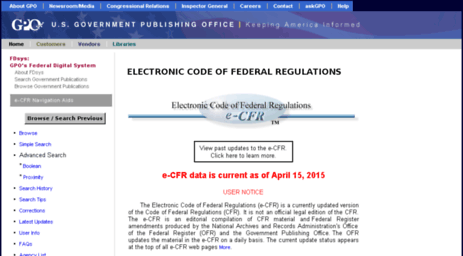The image appears to be a screenshot of a website that has been scaled down, making much of the text difficult to read. 

At the top of the webpage, there is a light blue navigation bar featuring white text links aligned to the left. These links include "About GPO," followed by a vertical line separator, then additional links for "Inspector General," "Careers," "Contact," "Ask GPO," and "Help."

Below the navigation bar, a thicker line is present, containing an image of the American flag and the GPO (Government Publishing Office) logo. In white font, it states "US Government Publishing Office." Beneath this is a yellow line with the tagline "Keeping America Informed" positioned towards the left.

Under this section, there is a gray box listing different categories: "Home," "Customers," "Vendors," and "Libraries," each in distinct colored fonts.

The main content area of the screen is divided into two sections. The left section features various menu options such as "Browse" and "Search Tips." The right section displays selected content. In this instance, it shows the title "Electronic Code of Federal Regulations" in bold black text next to a logo. Below this, there is a box prompting users to "View past updates to the ECFR" with a clickable link to learn more. Additionally, a paragraph underneath explains a user notice.

The remainder of the screen is occupied by a large black box, which likely contains additional website content or imagery that is not specified in the description.